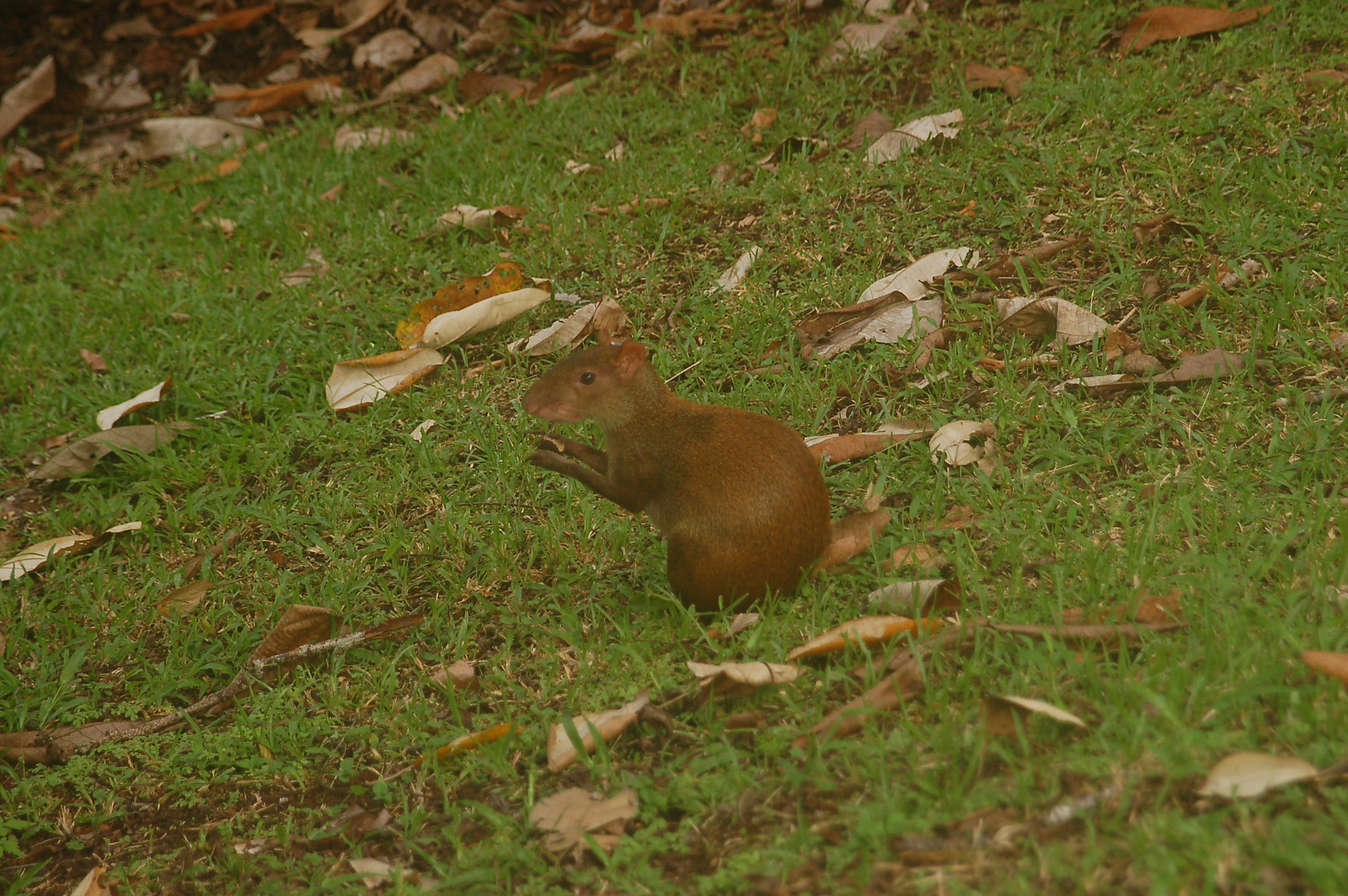In this detailed photograph taken outdoors, a small rodent, possibly a rat or mouse, is situated in the center of lush, green grass. The rodent features uniformly brown fur with a slightly darker face, and it is captured in a posture indicating it is eating, holding what seems to be a nut or seed in its clasped paws. Its alert demeanor is highlighted by one beady black eye facing the camera. The grass appears fresh and vibrant, suggesting recent rain, and while mostly covering the ground, allows glimpses of dirt beneath. Scattered brown leaves are evident throughout the image, curling and wilted, with a heavy concentration in the top left corner forming a dense pile where the grass is almost completely obscured. The rodent's body exhibits a thick, robust back half contrasting with its skinnier arms, and its head appears more mouse-like, lacking a bushy tail but with a larger, squirrel-like body. The creature sits on its hind legs, looking slightly to the left side of the photograph, giving an impression of attentiveness amidst its natural surroundings.